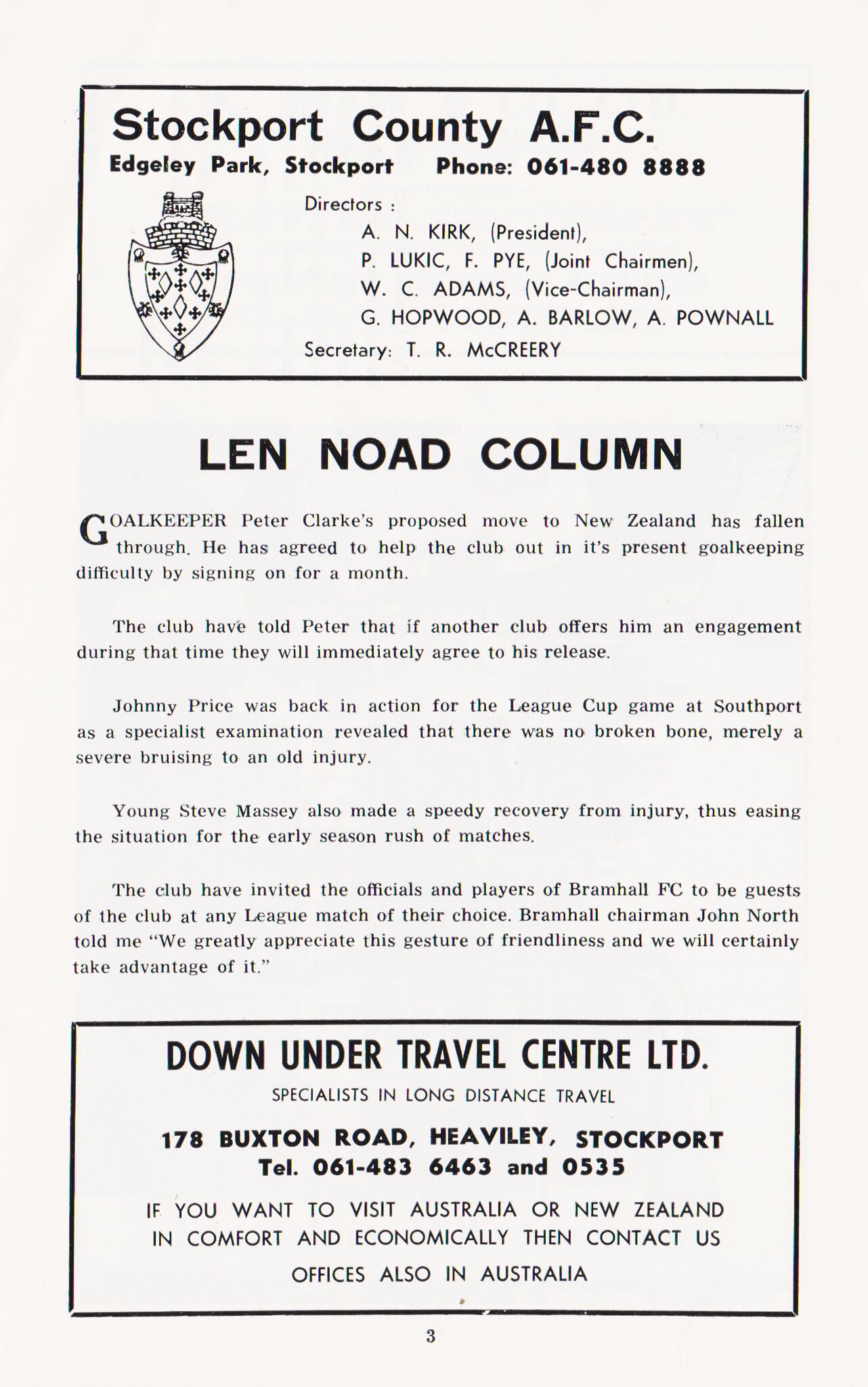A detailed page from a soccer publication, most likely a game day program or magazine, prominently features an advertisement on a plain white background with black text. The top section, enclosed in a black rectangle, is titled "Stockport County AFC, Edgeley Park, Stockport," and includes a phone number alongside a list of directors and a secretary. Adjacent to the list is the emblem of Stockport County. Below, the main body of the page features an article titled "Len Noad Column," which discusses the latest news regarding the football team in several short paragraphs. At the bottom of the page, there's another black-bordered box that serves as an advertisement for the "Down Under Travel Center, LTD," a specialist in long-distance travel. The ad promotes travel to Australia and New Zealand in comfort and economically, providing an address and phone number for more information. This layout is noted to be on page three of the publication.